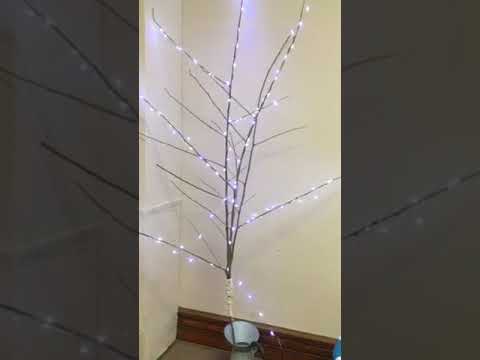The image is a square, artistic rendering featuring a central tree branch that splits into three main parts and has various smaller twiglets, all devoid of leaves. The branch appears to be a minimalist or makeshift version of a Christmas tree, adorned with tiny, glimmering white lights that give it a whitish glow, although the lights appear purple in some descriptions. This branch is set in a small vase or pot resting on a surface that looks like dark wood, possibly mahogany. The background consists of a light beige wall with shadows and a darkened vertical border on either side, giving the impression of a shadow letterbox effect. The scene appears to be captured indoors, with brown wooden flooring extending from the base.